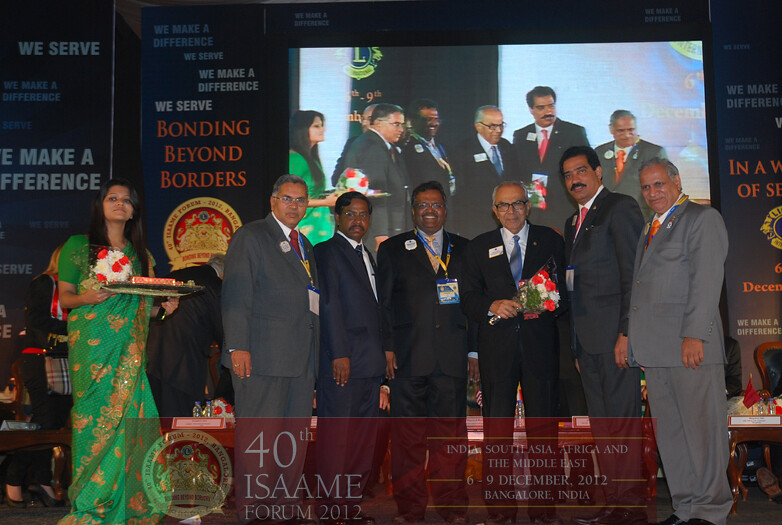The image captures a formal group photograph on a stage, featuring several men and one woman. The woman, positioned farthest to the left, is dressed in a light green and gold-patterned dress. She has long black hair and is holding a tray with her head slightly tilted up and mouth closed. Next to her are six men in suits of various colors—gray, dark blue, and black. The man immediately to her right is dressed in a gray suit with a red tie and brown skin; he wears eyeglasses, a lanyard with a white card, and has gray hair. Moving to the right, the next man also wears glasses, a black suit, and a white shirt with dark black hair and a closed mouth. The subsequent man is similarly attired in a black suit but with a blue shirt and gold tie; he is smiling, has eyeglasses, a lanyard, and a white badge on his upper left shoulder. Central to the group is a man with gray hair, glasses, and holding a bouquet of red and white flowers. He is dressed in a black suit with a white shirt and blue tie, with a white badge on his chest. The tallest man further to the right has a black mustache, black hair, and is wearing a dark suit with a red tie. The final man on the farthest right is wearing a gray suit, a white shirt, and has gray hair.

Behind them is a large projection screen displaying the event with advertisements surrounding it. The advertisements include the message "Bonding Beyond Borders" on an orange background and the phrases "We make a difference. We serve" on a dark blue backdrop. At the bottom of the image is a semi-transparent bar with the text "40th ISAAME Forum 2012, India, South Asia, Africa, and the Middle East, 6-9 December 2012, Bangalore, India" emblazoned upon it. The screen and text add context, indicating that this photograph was taken during a significant event, possibly involving award presentations or recognitions.